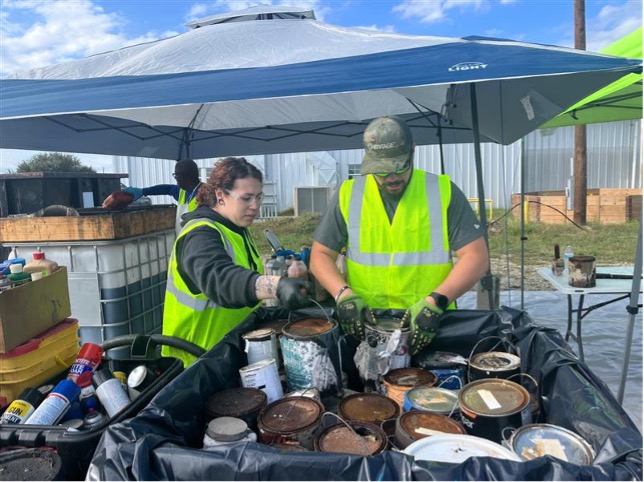In this landscape-oriented photograph, two Caucasian individuals, a man and a woman, are at the forefront, deeply involved in an apparent paint recycling project. The man, positioned on the right, wears a camo hat, glasses, and facial hair, along with a blue t-shirt under a yellow and silver safety vest. The woman, on the left, has brown hair, and she is dressed in a long-sleeve black shirt under a similar safety vest. Both are equipped with gloves and are leaning over a large tub filled with various paint cans, appearing to sort through them.

To the left of this tub is another container holding an assortment of spray bottles. In the background, a blue and gray umbrella offers some shade, punctuating the outdoor setting that features blue sky, grass, and trees. A third individual, another man in a safety vest, can be seen further back, standing at a multi-colored countertop, also engaged in sorting or organizing materials. The scene suggests an organized effort to dispose of or recycle paint responsibly.